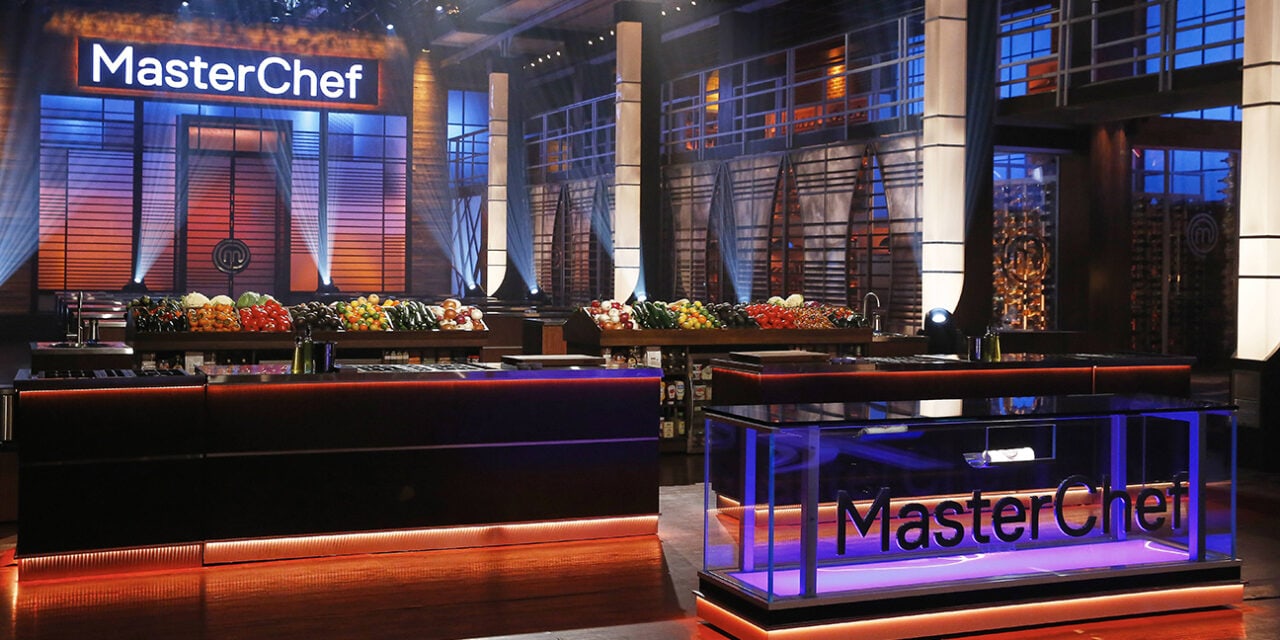The image captures a dramatically lit set of the reality television show MasterChef, renowned for its competition among amateur cooks aiming for a recipe book deal. Central to the set's design are multiple stylized kitchen stations, resembling black boxes adorned with glowing LED lights and brown wooden bases, equipped with sinks, stoves, and ovens. Behind these stations, shelves brimming with fresh produce like cucumbers, mangoes, tomatoes, and lemons, as well as condiments, wines, and olive oils, provide a vibrant backdrop. The set features the MasterChef logo prominently in large white letters, both above a doorway and within a glass-framed table at the judges' podium, which is illuminated with blue and purple lights. This podium, potentially containing a white apron, marks the place where contestants present their dishes. The expansive, studio-like kitchen also includes elements such as a second-floor balcony with light columns and a railing, enhancing the dramatic, high-end aesthetic crafted for television.